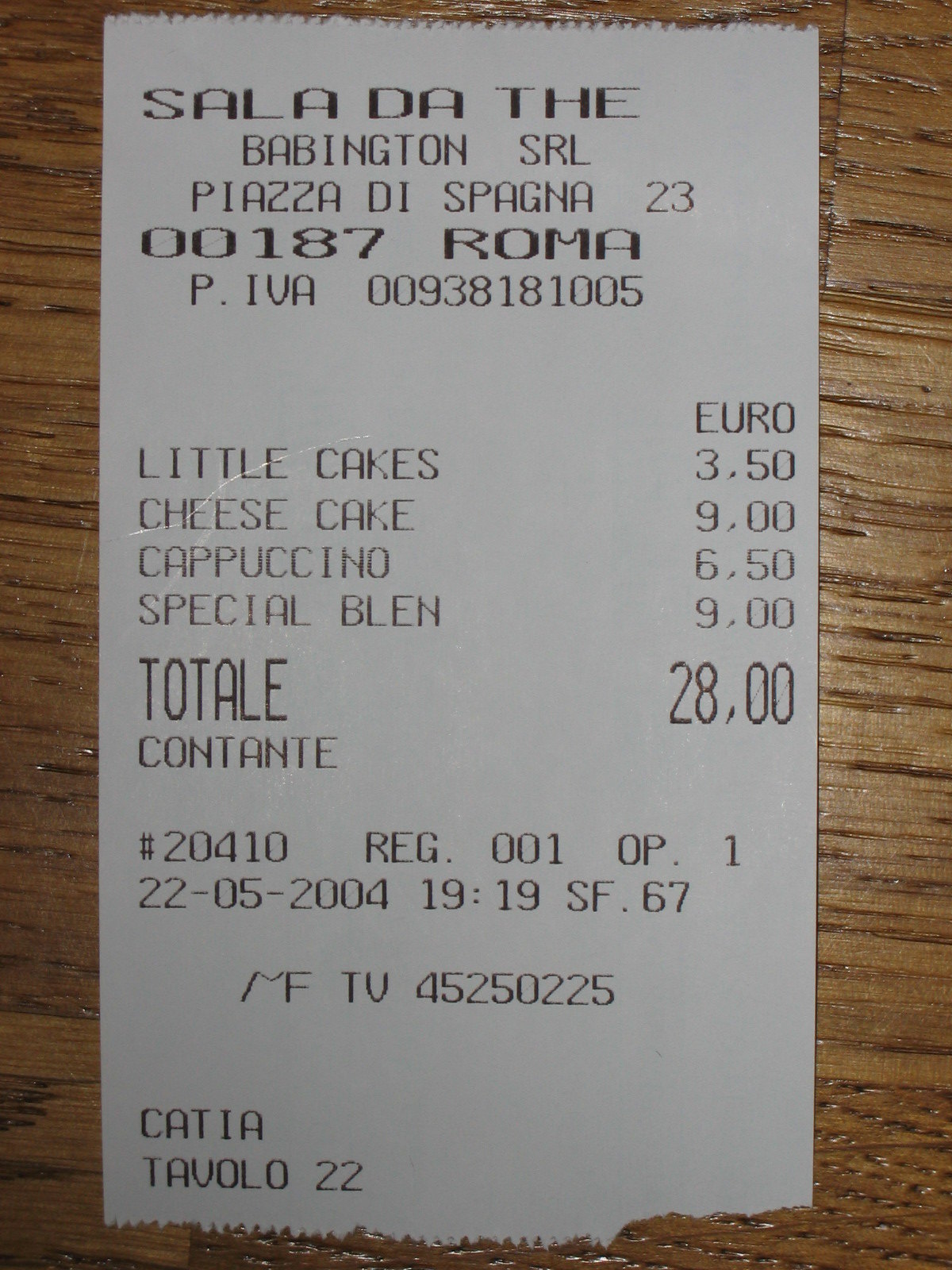The image displays a photograph of a white receipt from a grocery store named "Salada," likely located in Rome, Italy. The receipt's header prominently features "Salada" and "Babington SRL," followed by the address "Piazza di Spagna 23, 00187 Roma." Below this, it includes the VAT number "P.IVA 00938181005." The listed items indicate purchases of little cakes (€3.50), cheesecake (€9.00), cappuccino (€6.50), and a special blend (€9.00), totaling €28.00. Additional details on the receipt include numerical codes such as "20410, REG001, OP1," a date "22-05-2004," and a time "19:19." Near the bottom, phrases like "SF67" and the number "FTV45250225" are visible. The receipt ends with "Catia Tavola 22," which likely translates to "Table 22" in Italian. The receipt rests on a wooden surface with a horizontal grain pattern.